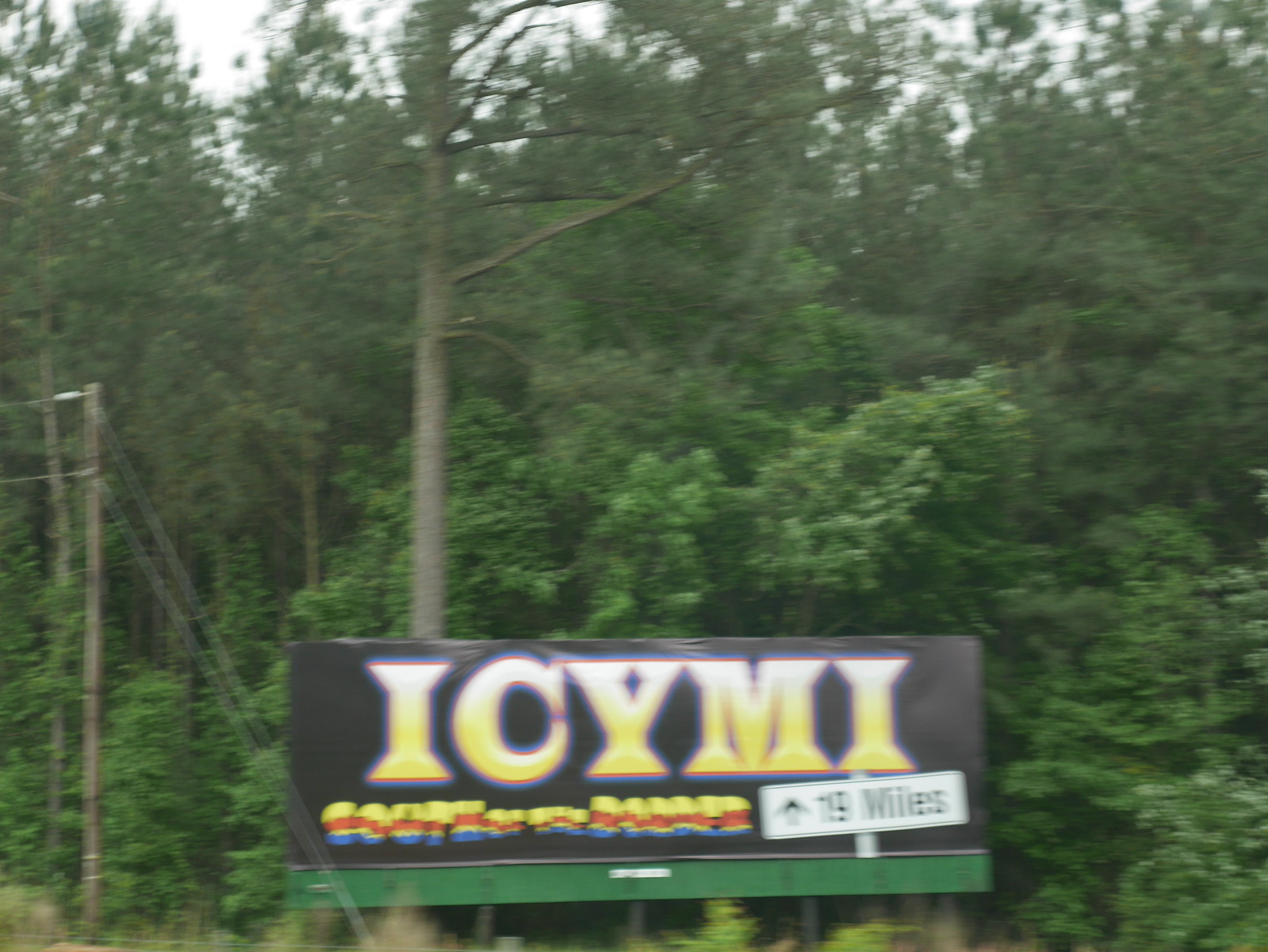In the foreground, there is a low-level rectangular billboard standing prominently against a vibrant backdrop of tall trees, all adorned with lush green leaves that extend beyond the frame. The tallest tree immediately behind the sign towers so high it disappears from view. On the left side of the image, a brown pole with two wires draped across resembles a telephone wire, adding a touch of urbanity to the natural scene.

The billboard itself is distinctly black with mostly yellow and white lettering. Dominating the sign are the bold, capital letters "ICYMI" in yellow, transitioning to white at the top. Below this, a smaller, blurred word in red, white, and blue is partially legible even when zoomed in. Adjacent to this sign is another straightforward sign stating "19 miles" accompanied by a straight-ahead arrow in black.

This juxtaposition of modern signage amid the tranquil, towering forest creates a striking visual contrast.